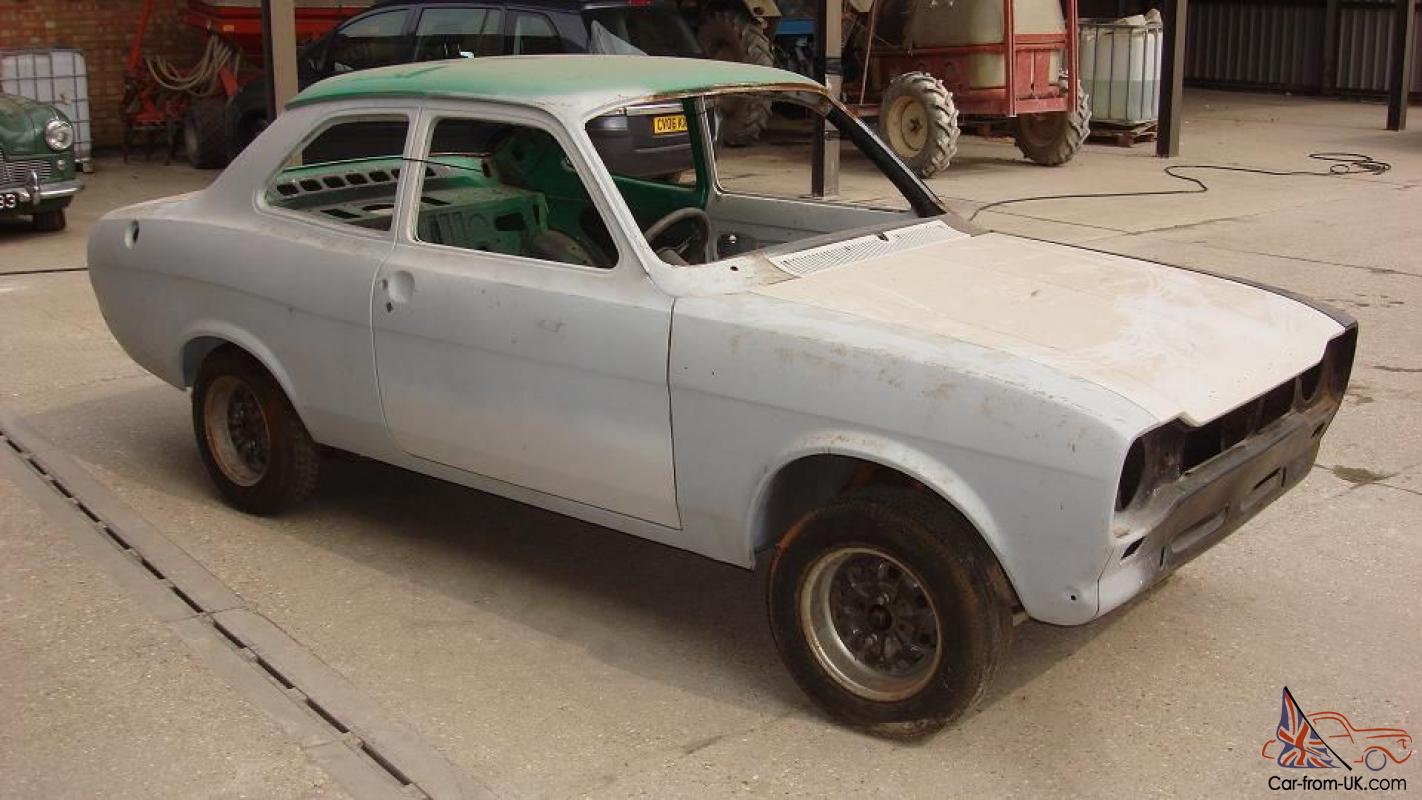The photo captures a worn-out 1960s or 1970s two-door sedan parked diagonally in the center of an expansive garage or workshop. The car's light gray and greenish paint is severely faded, revealing patches of beige and white. It lacks both the bumper and headlights, and the tires, though present, are worn out with no hubcaps. The interior is stripped down to metal and is missing the seats and door handles. The scene around the car includes a large open garage space with brown poles, cords strewn across the floor, and other old vehicles, including a tractor, in the background. A logo in the lower right corner bears the text "car-from-uk.com" in red line art, featuring an image of a car with the UK flag. The setting is well lit, suggesting the work is indoors despite the open, airy feel. The picture’s color palette includes shades of green, gray, red, white, blue, black, yellow, and beige, contributing to the overall sense of an old vehicle awaiting restoration amidst a cluttered yet resourceful environment.